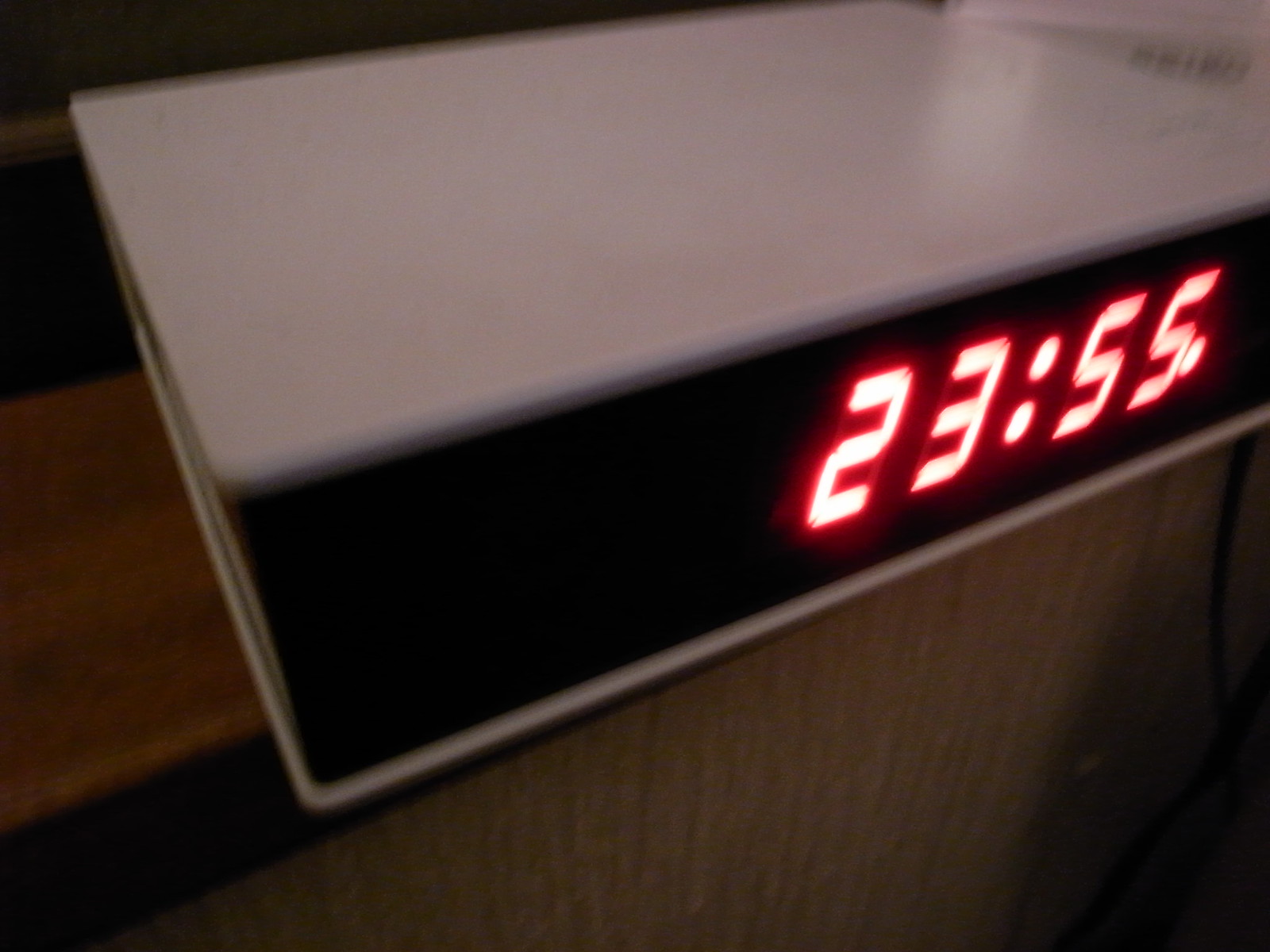The image depicts a digital clock displaying the time "23:55" in bright red numerals. The clock's design features a black face, contrasting with its white top and bottom surfaces. Positioned on a wooden surface, possibly an end table or nightstand, the clock evokes a sense of a bedroom setting, though this isn't confirmed. A black power cord is slightly visible on the far right of the image, casting a shadow beneath it. The absence of additional icons or markings suggests that this is a simple, straightforward clock, primarily serving as a timekeeping device.